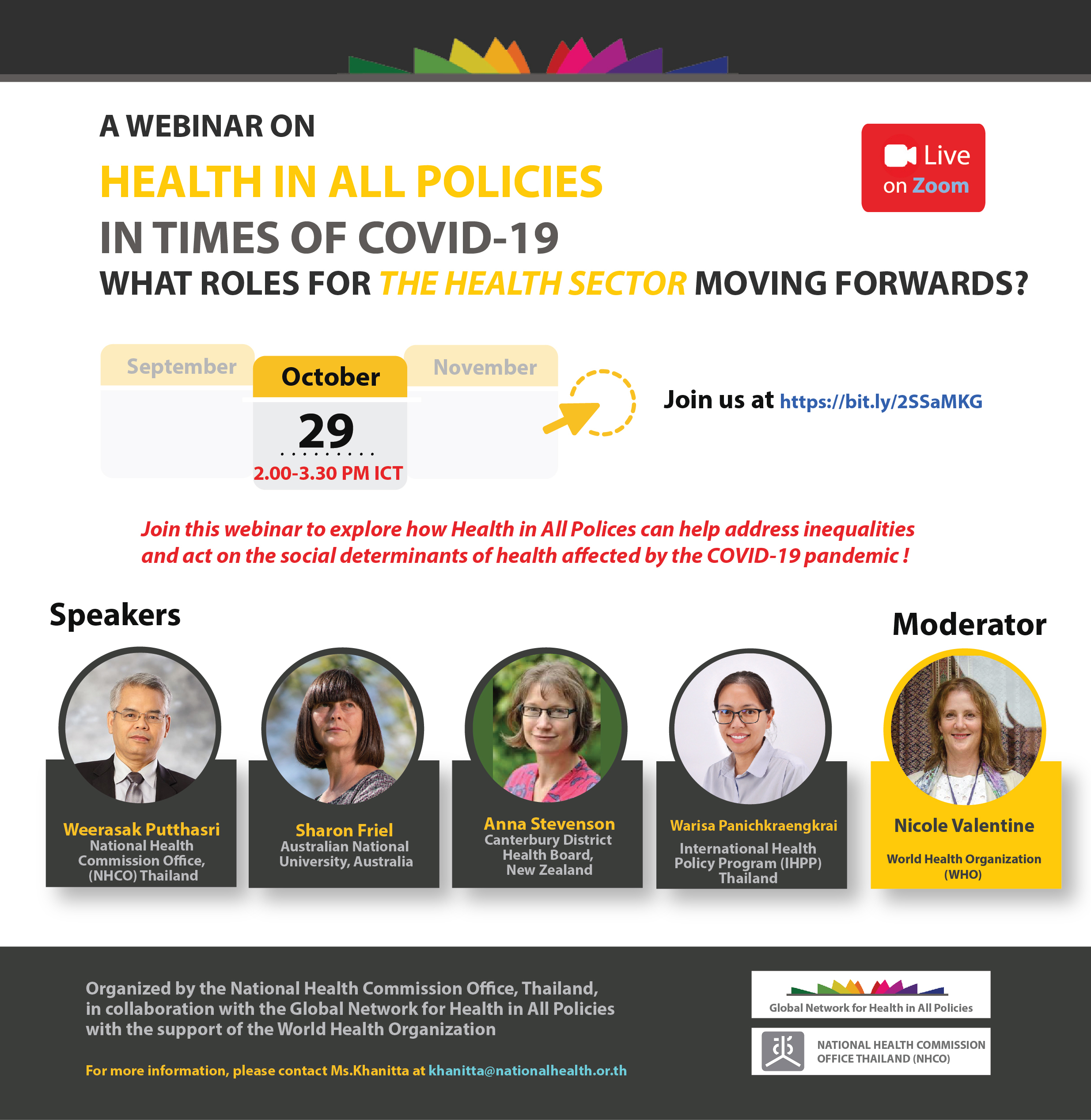The screenshot is from a website promoting an upcoming webinar, featuring a detailed and colorful layout designed to attract attention. At the top, a black border is adorned with a striking series of rainbow-colored triangles, transitioning smoothly from dark green on the left to dark blue on the right.

Beneath this vibrant border lies the webinar's header on a clean white background. It starts with the text "A Webinar on" in sleek black font. Highlighted in bold yellow text just below, the main focus of the webinar is revealed: "Health in All Policies." Further descriptive text in black reads, "In times of COVID-19: What roles for," followed by "the health sector" in yellow and concluding with "moving forwards" in black.

An informative image displays the event's timing: October 29th, from 2:00 to 3:30 p.m. ICT. The call to action follows, prompting potential attendees to join via the provided short URL: "https://bit.ly/2SSAMKG."

In red text, the webinar's purpose is emphasized: "Join this webinar to explore how Health in All Policies can help address inequalities and act on the social determinants of health affected by the COVID-19 pandemic."

Below this engaging introduction is a series of images featuring all the speakers, complete with their names. The layout culminates with an image of the moderator, Nicole Valentine, positioned on the far right, underscoring her role in guiding the upcoming discussion.